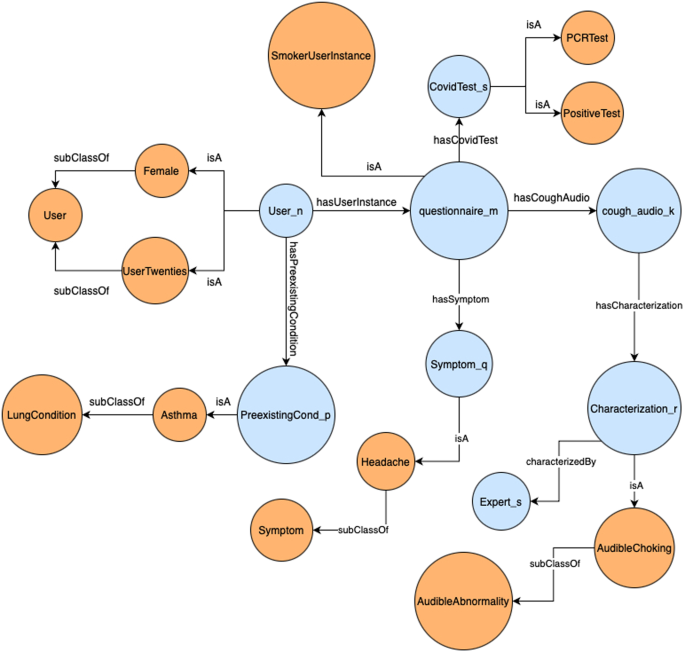The image presents a detailed flowchart on a solid white background featuring multiple interconnected circles, outlined in black, with varying sizes and colors. At the center top, there is an orange circle labeled "Smoker User Instance," which serves as a focal point. Throughout the diagram, circles are connected with arrows, each labeled to specify the type of relationship. 

To the upper right of the central circle, there is another orange circle labeled "PCR Test," followed by a smaller circle beneath it named "Positive Test." Between these orange circles are a series of blue circles, including one labeled "COVID Test," directly below which are blue circles labeled "Questionnaire M" and "Symptom Q." 

On the image's left side, a small section forms a rectangular structure composed of interconnected circles with arrows. The left circle in this section is labeled "User," the top circle is "Female," and the bottom circle reads "User 20." Other noteworthy blue circles spread across the left of the diagram include labels like "Cough Audio K," "Characterization," and "Symptom Q."

Additional blue circles are labeled "Questionnaire M," "User N," "Characterization R," "Export S," and "Pre-Existing Condition P." The orange circles interspersed through the diagram include labels such as "Audible Checking," "Talking," "Audible Abnormality," "Headache," "Symptom," "Asthma," and "Lung Condition." 

Arrows between the circles bear labels that describe relationships and actions such as "Has Symptom," "Has Characterization," "Subclass Of," and "ISA." This detailed layout illustrates the interconnectedness of various health-related instances and states in a structured visual format.